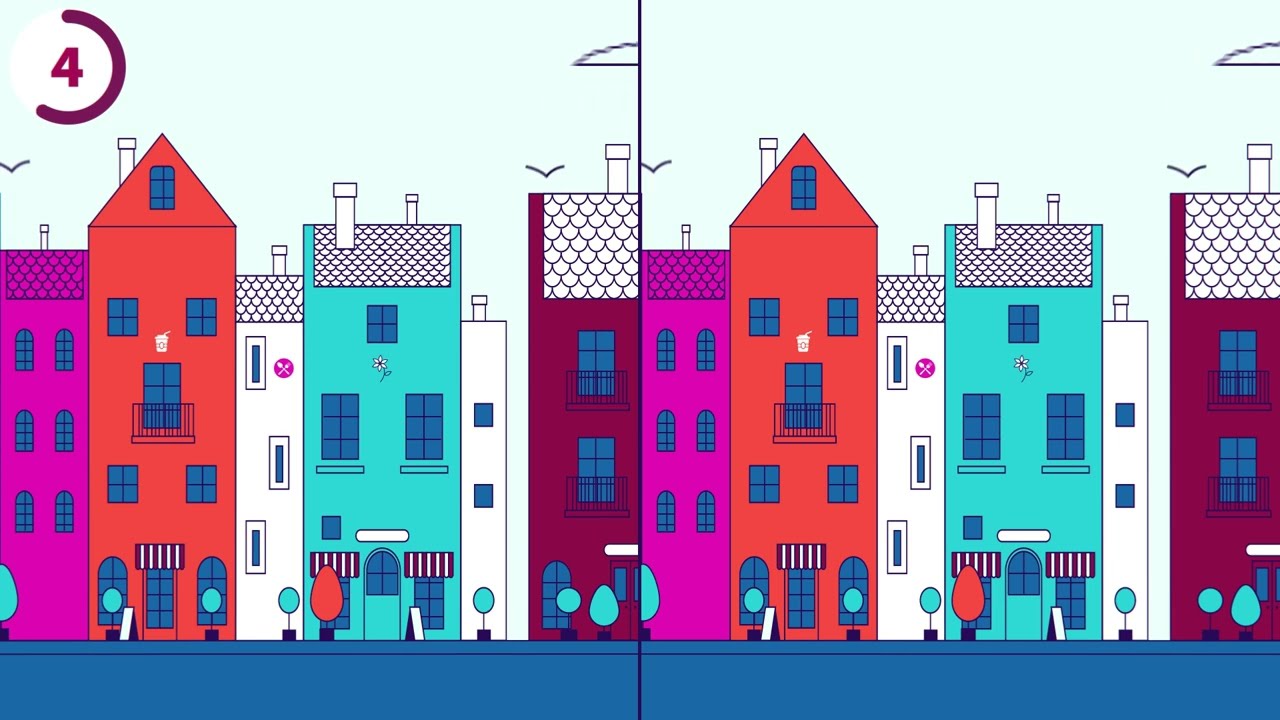This image is a detailed, side-by-side mirrored line drawing of a series of colorful buildings from a small town, split by a vertical black line at the center. The duplication indicates a spot-the-difference type of game, suggested by the presence of a red number four within a half-outlined maroon and white circle in the upper left corner. The buildings, each at least three stories high, present in vivid hues. Starting from the left, a tall, thin fuchsia building with blue arched windows and a flat roof is followed by a red building with a unique arched roof and blue rectangular and square windows. Third is a narrow white building with a flat roof and three rectangular windows. Next is a slightly broader light blue building with a flat roof, two chimneys, and more rectangular windows, adjacent to a very thin white building featuring two square windows and a single chimney. There is a noticeable gap before reaching the last, wider maroon building with two blue rectangular windows and a singular arched window at the bottom. The lower part of the image includes a blue road lined with teal-colored trees that have round bush-like tops, along with a distinctive red egg-shaped tree. In the sky, a few clouds are scattered, and birds are flying. Each visual element is mirrored on the right-hand side, making the drawings identical save for the timer in the upper left corner.